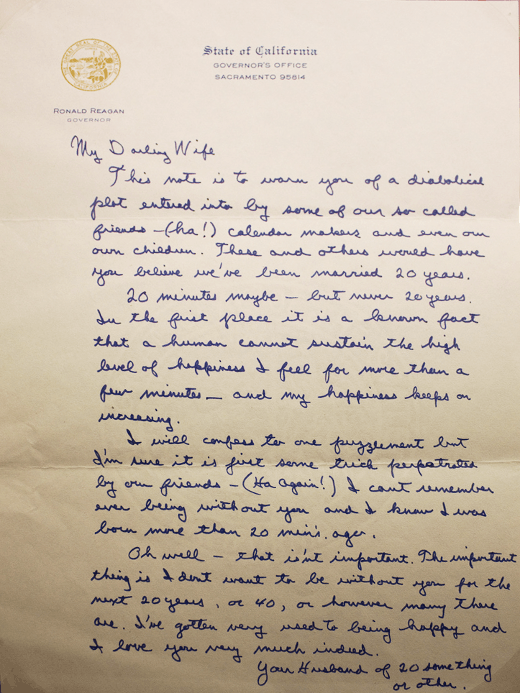The image shows a handwritten letter that displays the age and wear of time, with the paper itself having turned a brownish-yellow color. The letter, composed in blue ink, hails from the Governor's Office of the State of California, specifically Sacramento, zip code 95814. In the top left corner, there's a notable stamp – the official state seal – beside which is inscribed the name "Ronald Reagan, Governor," indicating the letter was penned during Reagan’s tenure as governor. The letter opens with an affectionate greeting, "My Darling Wife," revealing it is addressed to Reagan’s wife, Nancy. The contents intriguingly mention a warning about a diabolical plot by some friends, punctuated with a light-hearted "Ha!" The exact authentication of the document is unclear, but its personal nature and cursive script offer a charm rare in contemporary correspondence.